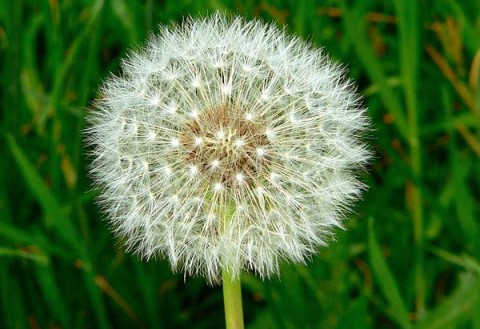In this high-definition, close-up photograph taken by a skilled photographer, the primary focus is on a single white dandelion, the kind traditionally used for making wishes. The image is rectangular, wider than it is tall, and meticulously brings out the intricate details of the dandelion, from its brown central core to the delicate white tendrils that form a perfect circular shape. This dandelion stands out clearly against a blurred background of tall, vibrant green grass mixed with some brown, with the dandelion's lighter green stem providing a contrasting touch. The overall composition beautifully highlights the ethereal and wispy nature of the dandelion, capturing its fleeting elegance amidst the lush, slightly faded foliage.